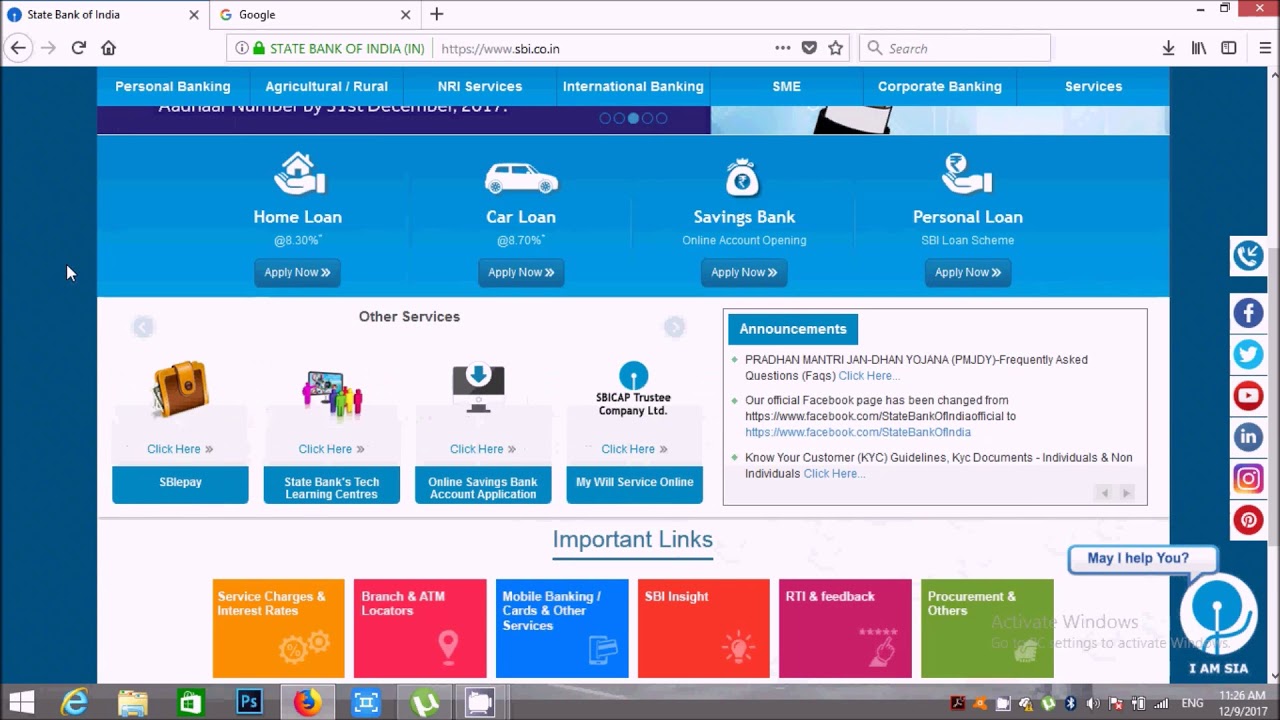A screenshot of a web browser window showcasing the homepage of the State Bank of India (SBI) website, viewed using Firefox on a Windows computer. The recognizable Windows logo is visible at the bottom left corner of the screen, confirming the operating system. At the top left of the browser, the State Bank of India's name is prominently displayed in green, next to a green padlock symbol, indicating a secure connection (https://www.sbi.co.in).

The browser shows two open tabs: one for the SBI homepage and another for Google. The address bar confirms the site's legitimacy with the secure URL mentioned. The homepage features a dark blue background with a mid-blue menu bar that contrasts with white text, providing clear navigation options. These options include "Personal Banking," "Agricultural/Rural," "NRI Services," "International Banking," "SME," "Corporate Banking," and "Services."

Prominent on the page are several icons representing different services: a hand holding a house for "Home Loan" with an "Apply Now" button, a car for "Car Loan" also with an "Apply Now" button, and options for "Savings Bank" and "Personal Loan." Beneath these icons, there's a series of colored rectangles offering quick links to various other services such as "Service Charges and Interest Rates," "Branch and ATM Locators," "Mobile Banking/Cards and Other Services," "SBI Insight," "RTI and Feedback," and "Procurement and Others." The overall design uses a blue theme for a cohesive and professional appearance.